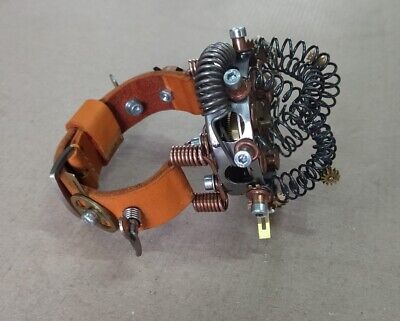The image depicts a peculiar mechanical device set against a flat, gray background, potentially concrete. On the left side, the device features a thick, orange leather strap, resembling a bracelet, adorned with numerous dials, screws, and controls. An additional small leather piece encircles the strap, which is fastened to the right-side component by two tightly wound bronze-colored coils.

The right-side component, partially revealed, consists of stainless steel and is cluttered with various metal springs of different states – some tightly coiled, others more relaxed. This area also includes several screws securing the springs in place. The right section appears chaotic with its black, tangled springs, contrasting with its sleek metallic construction. Together, these elements blend into a unique and complex machine.